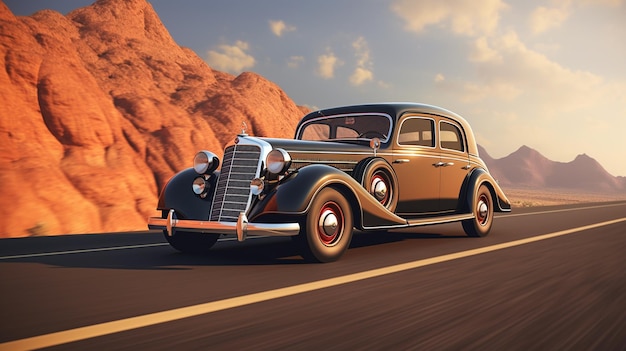A digital artwork showcases a black, vintage Mercedes-Benz traveling down a beautifully depicted American highway, set against a backdrop of realistic-looking Redstone Mountains. The car, which features distinctive chrome on the front and hubcaps, as well as four central headlights and an iconic Mercedes logo, appears to be from the early to mid-1900s. The scene captures a radiant blue sky adorned with realistic clouds and the sun lighting up the eastern side, casting the car's shadow on the road. The road itself is detailed with streaked pavement, a central yellow line dividing the two lanes, and a white line marking the edge. Although the car is equipped with a spare tire by the driver's side door, an intriguing detail is the apparent absence of a driver.